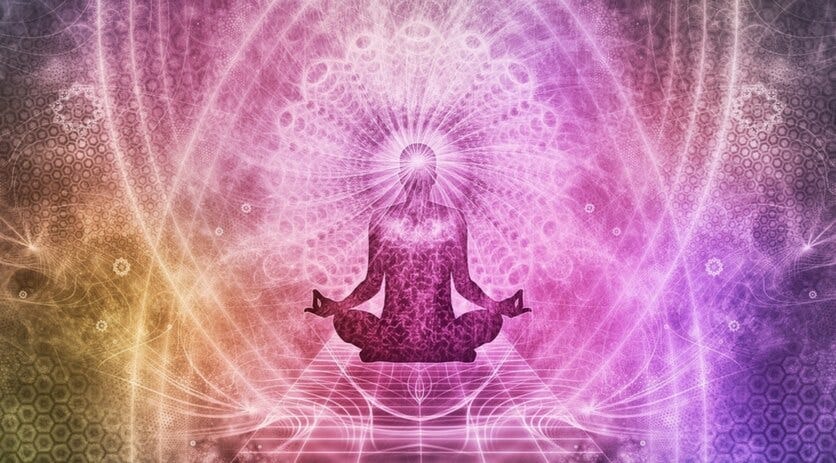This captivating artistic illustration features a purple silhouette of a person seated in a cross-legged, meditative yoga pose, with their fingers in the "on" position and their wrists resting on their knees. The figure is positioned on a geometric plane or grid that extends outwards from the center bottom of the image to just past the silhouette, emphasizing the serene and grounded nature of the pose. Intricate geometric shapes, including hexagons, circles, and curving lines, swirl around the figure in a mesmerizing circular pattern, with ever-smaller patterns converging around the person's glowing head. The predominant colors of these patterns are white and silver, creating an ethereal and otherworldly aura around the individual. The background is a rich tapestry of colors, with hues of gold and brown at the bottom left transitioning through pinkish purple and darker purple, culminating in black and dark blue in the upper corners. Light beams emanate from the center of the figure's head, radiating outward in staggered ovals, adding to the psychedelic ambiance of the piece. This image beautifully blends elements of meditation, spirituality, and geometry, enveloping the viewer in a cosmic and transcendental experience.